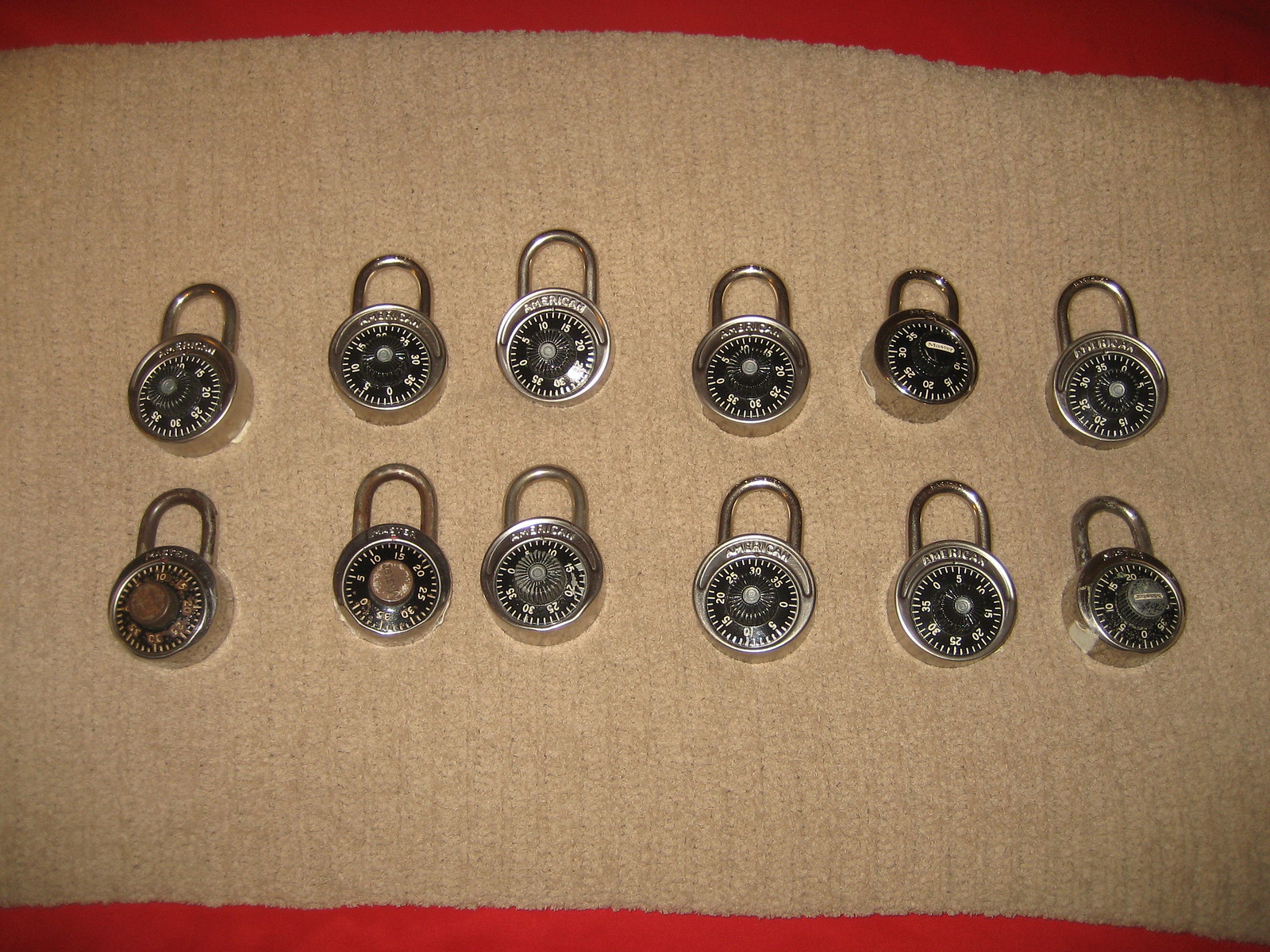This photograph captures 12 combination locks arranged in two rows of six on a brown blanket, which itself is placed on a backdrop of a reddish table or floor. The locks, predominantly uniform in design, feature black circular dials with white numbers on stainless steel bodies. While most of the locks are shiny and look unused, two in the bottom left corner appear rusty and worn, suggesting different usage histories or eras of production. There's also a unique brown lock situated as the first in the bottom row on the left-hand side, standing out amidst the otherwise black dials. The alignment of the locks is slightly irregular, adding a natural, unposed feel to the image.